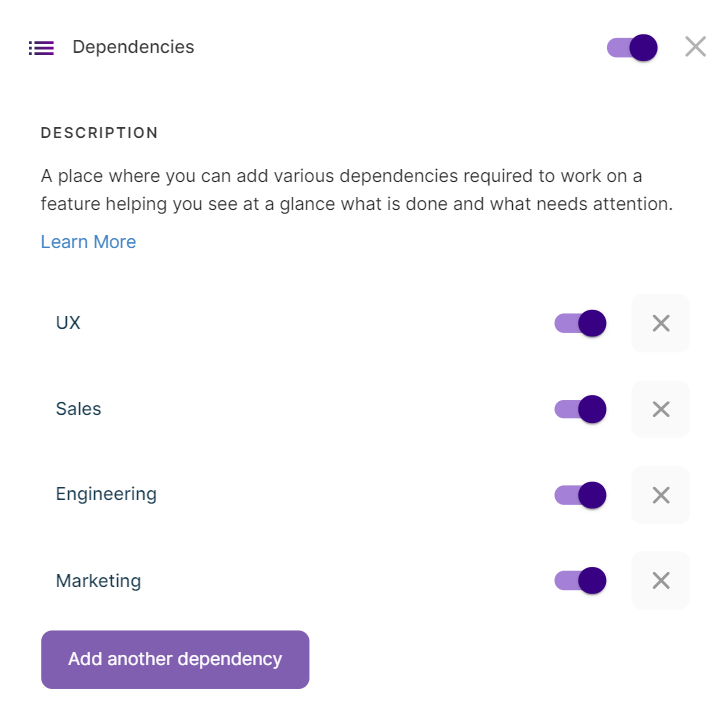Screenshot of a Settings Page for Managing Dependencies

The screenshot depicts a settings page designed for managing various dependencies essential for working on specific features. Located at the top left corner, a hammer icon provides navigational options within the site. Adjacent to this icon, the word "Dependencies" is prominently displayed, indicating the section being viewed. A status indicator to the right of "Dependencies" shows that the dependencies feature is currently turned on.

Beneath the heading, a section labeled "Description" explains that this area allows users to add and monitor different dependencies required for feature development, offering a clear overview of completed tasks and areas needing attention. An option to "Learn more" is provided for additional information.

The page lists four dependencies, each with a toggle switch to enable or disable them:

1. **UX** - Enabled
2. **Sales** - Enabled
3. **Engineering** - Enabled
4. **Marketing** - Enabled

At the bottom left corner, a prominent purple button labeled "Add another dependency" invites users to input and manage new dependencies as needed, enhancing the functionality and customization of the workspace. The context suggests that this page is likely part of a management tool for a website or application development environment, given the nature of the dependencies listed (UX, Sales, Engineering, and Marketing).